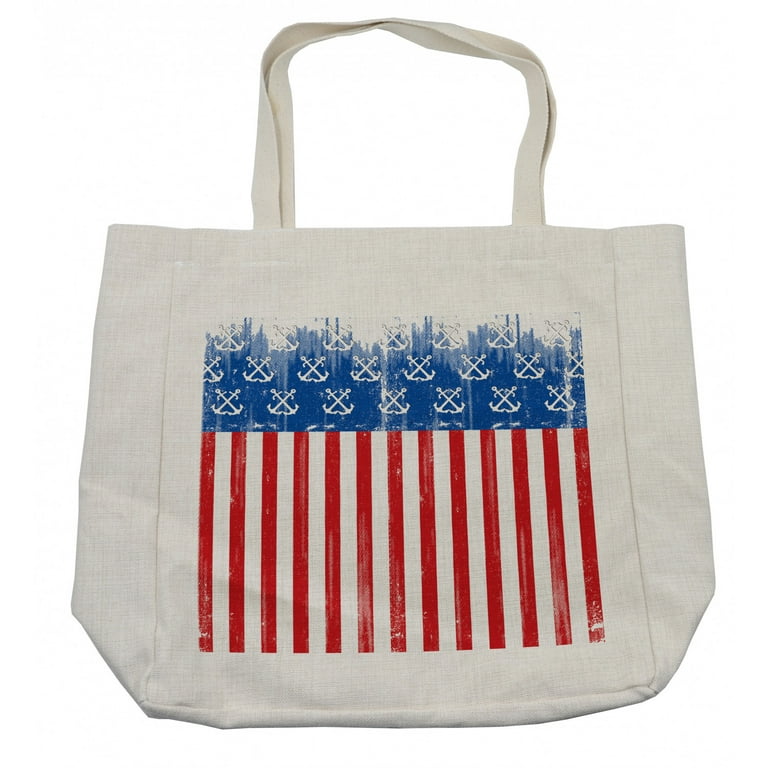The image features a light tan canvas tote bag with a distinctive American flag-inspired graphic on the front. The bag is primarily roundish with slight angled corners at the bottom left and right. Its two large white straps emerge from the top, providing robust support. The graphic at the center of the bag mimics a distressed, weathered American flag. The upper section of this graphic is a streaky blue background adorned with white anchors arranged in cross-like X patterns, replacing the traditional stars. Below the blue section, red and white stripes run vertically down the tote's front. The colors—light tan, white, red, and blue—are purposefully designed to appear worn and vintage, enhancing the bag's rugged texture. With no items inside, the tote bag lies flat against a plain background, suggesting it might be a product image for an online marketplace such as Etsy.